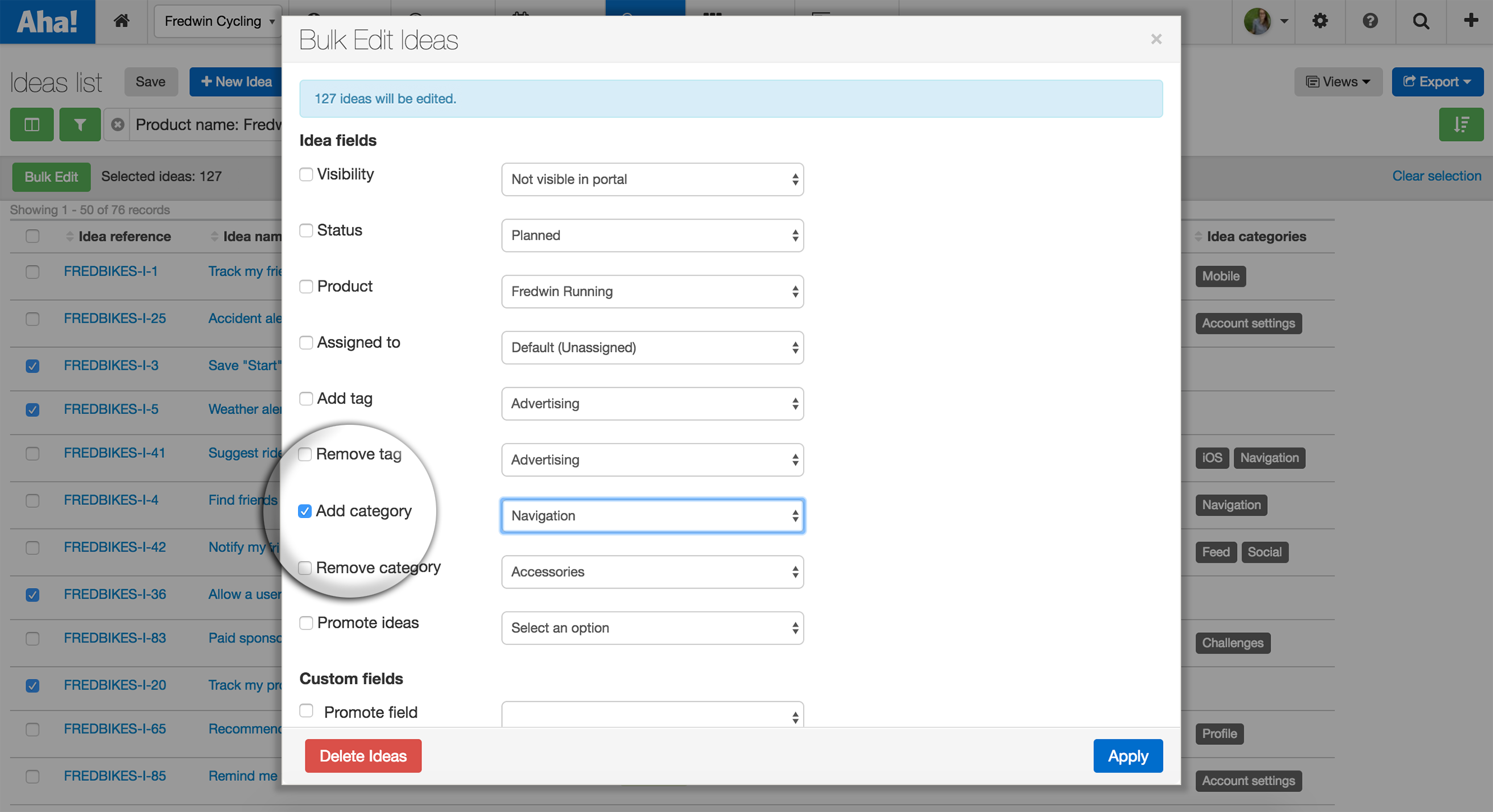This image displays a screenshot from a computer, showcasing an interface designed for bulk editing. A prominent rectangular dialog box has appeared on the screen, likely in response to a user's action. This box captures attention with a highlighted section labeled "Add Category" within a circled area for emphasis, accompanied by a magnifying glass icon to enhance visibility. The "Add Category" field is set to "Navigation" and is marked with a blue check mark, indicating it's selected.

At the top of the dialog box, a header reads "Bulk Edit Ideas," informing the user that 127 ideas will be edited in bulk. Below this header, a list of editable items is displayed in a column. Each entry includes a checkable square box next to it, currently showing as plain white squares that can be clicked to turn blue with a white checkmark. The editable fields are as follows: 

- Visibility
- Status
- Product
- Assigned To
- Add Tag
- Remove Tag
- Add Category (highlighted with a circle)
- Remove Category
- Promote Ideas

For the category "Visibility," the status is marked as "Not Visible In Portal." The "Status" category is set to "Planned." The field for "Product" reads "Fredwynn Running," while "Assigned To" is marked as "Default Unassigned." The "Add Tag" and "Remove Tag" fields are both labelled "Advertising." The "Add Category" field is set to "Navigation" (as emphasized with a circle), and the "Remove Category" field is labeled "Accessories." The "Promote Ideas" field has the option "Select An Option."

At the very bottom of this dialog box, a prominent red rectangular button with white text reads "Delete Items," suggesting an option to remove the selected entries. The overall interface appears organized and ready for the user to make bulk edits efficiently.